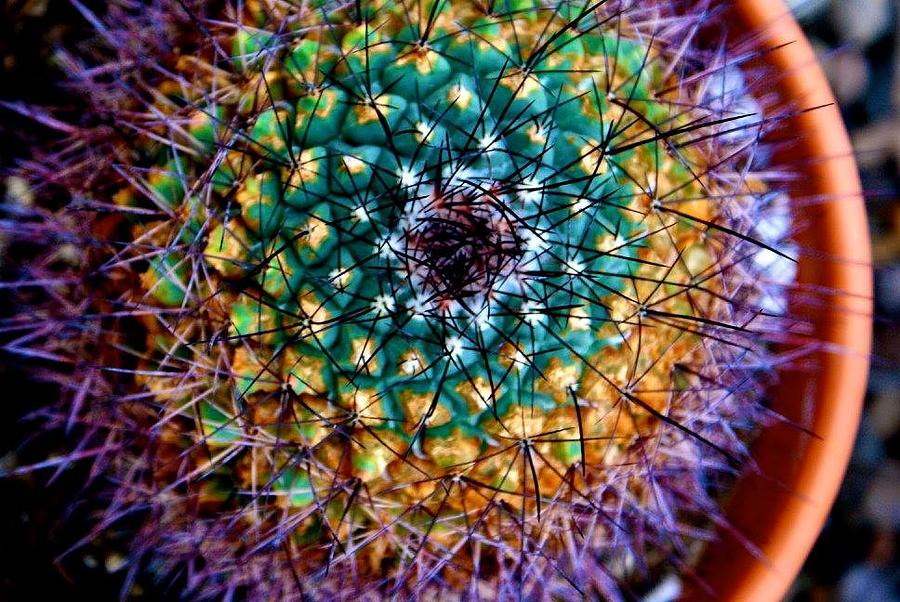The photograph is an extreme close-up, high-definition image of a cactus captured from above, resembling an aerial view. The brightly colored succulent appears to be photomanipulated to exhibit a psychedelic array of colors including bands of blue, red, green, purple, yellow, and teal, with some scattered white. The rim of the terracotta pot is visible in the background, subtly blurred to emphasize the cactus's vivid details.

The cactus's radiating pattern displays multiple rows of buds or protrusions from which black spikes emerge. The outermost ring of the cactus displays a beautiful shade of purple, transitioning to a pineapple-like texture and color, then shifting into turquoise, and finally converging back to purple at the center. This complex color pattern, combined with the sprigs of sharp cactus prickers, gives the impression of looking at an outer space formation or a textured, fuzzy eyeball. Despite its visually captivating appearance, the spiked surface hints at its prickly nature.